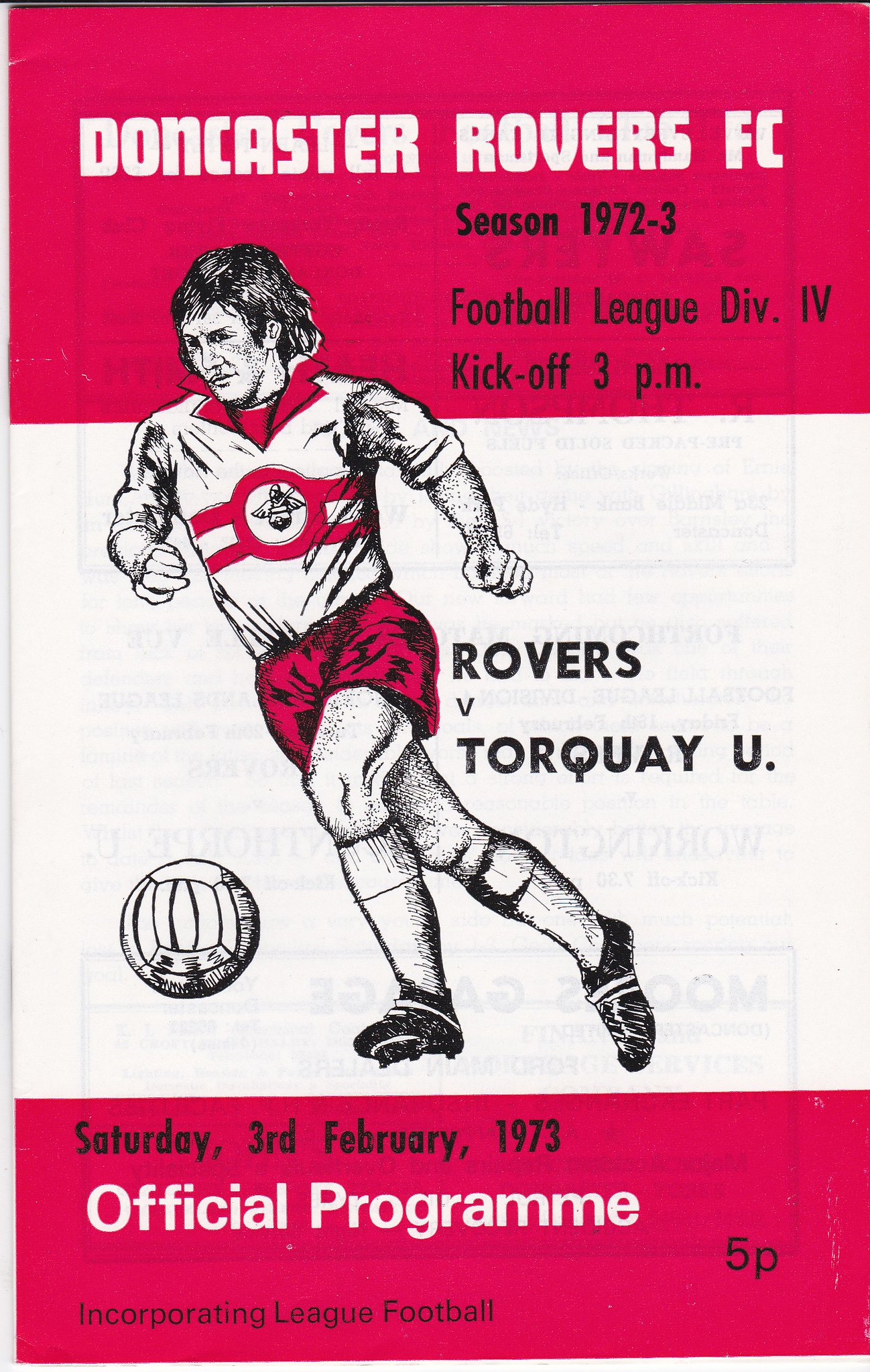This image from a 1972-73 Doncaster Rovers FC program guide page showcases a meticulously detailed vintage sketch of a football player poised to kick a soccer ball. The player is central to the composition, dressed in a white jersey with a distinctive red collar and a red emblem featuring the team's coat of arms. He wears matching red shorts and football shoes, with the sketch rendered in pen or pencil. The cover is marked by a red stripe at the top and bottom, enhancing its visual appeal. Key textual elements include "Doncaster Rovers FC, Season 1972-73, Football League Division 4, Kickoff 3 p.m., Rovers versus Torquay U, Saturday, 3rd February 1973," and "Official Program, 5p, Incorporating League Football," all styled in red, black, and white fonts. This evocative image is a snapshot of football history, encapsulating the essence of the era through design, style, and comprehensive program information.